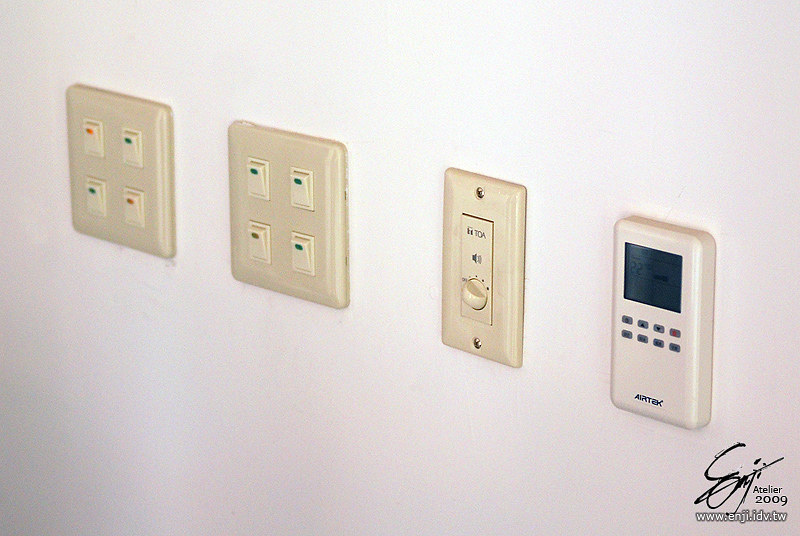The image depicts a section of a wall featuring several control panels and a thermostat. On the far left is a digital thermostat branded Airtek (A-I-R-T-E-K). The thermostat has an off-white, eggshell color and features a digital display along with eight buttons arranged in two rows of four. 

To the right of the thermostat, there are three plates on the wall. The first two plates each contain four switches, situated in each corner of the plate. The switches on the first plate are marked with colored dots in the following order: orange (top left), blue (top right), blue (bottom left), and orange (bottom right). The switches on the second plate are marked with blue (top left), blue (top right), brown (bottom left), and blue (bottom right) dots.

The third plate features a dial instead of switches. The dial has five notches indicating various levels, and it is currently set to the lowest point. The text above the dial is unreadable, making it unclear what the dial controls.

At the bottom right corner of the image, there is a watermark with a handwritten capital "S" followed by the word "ATLIER 2009" and the URL "www.engji.idv.tw".

Overall, the configuration suggests the presence of a mixture of light or other types of switches and a dial, possibly for controlling factors such as temperature or sound.